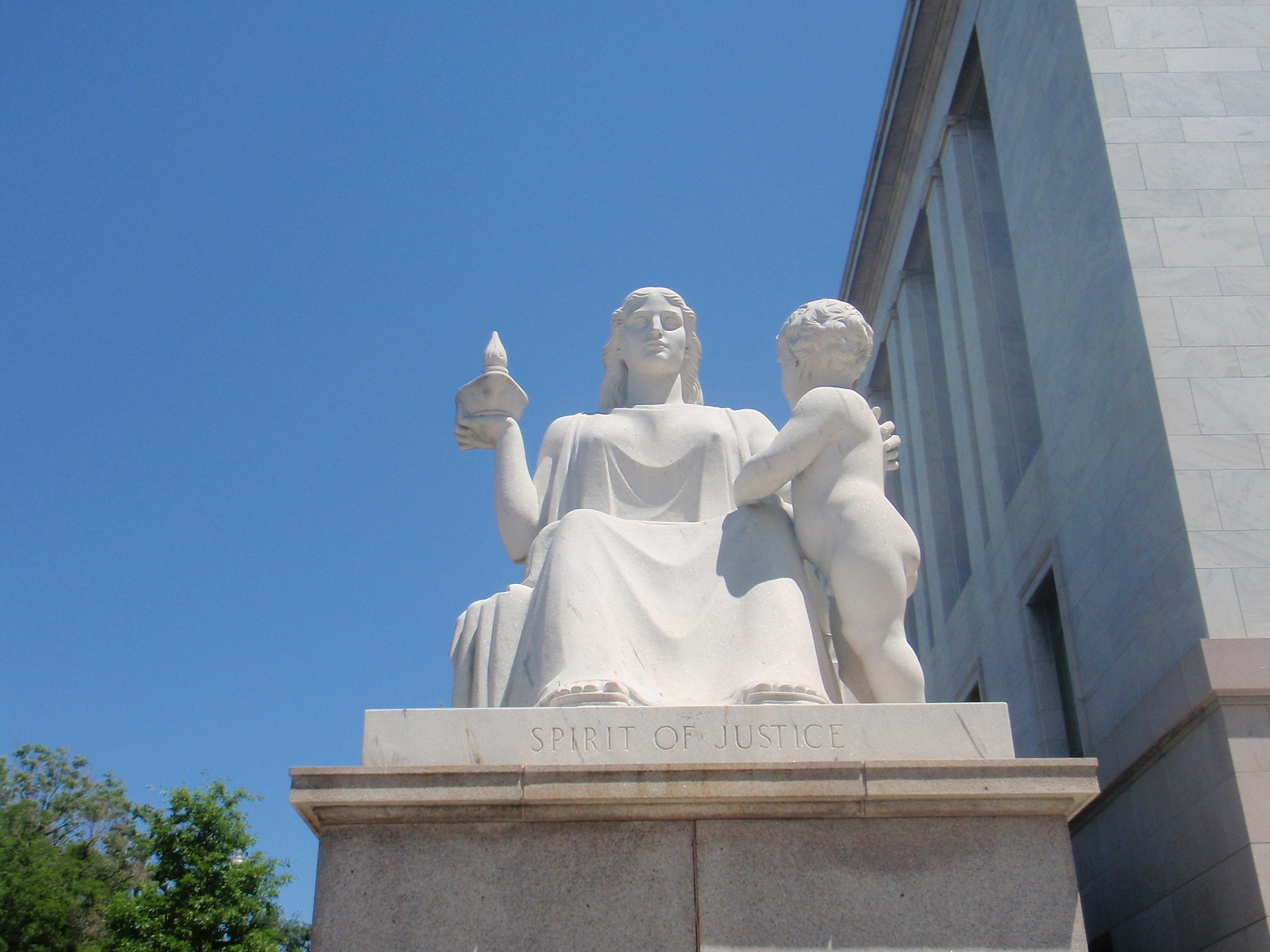The photograph captures a striking outdoor scene focused on a white statue, centrally placed in the frame. The statue depicts a woman with long hair, draped in a flowing garment, crafted from what appears to be stone, marble, or granite. She is holding a candle holder with a lit candle in one hand, while her other hand rests gently on the shoulder of a small, cherubic child who stands naked to her right, leaning against her knee. The child’s posture conveys a sense of comfort and protection. The base of the statue, made of a darker concrete or marble, bears the engraved text “Spirit of Justice.” Surrounding the statue, the left side features the green foliage of a tree, while the right side shows a tall, government-looking building against a backdrop of clear blue sky, devoid of clouds. The angle of the photograph suggests it was taken from slightly below eye level, emphasizing the statue's grandeur and the expanse of the sky above.